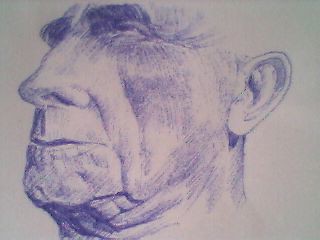The image is an ink sketch of an elderly man drawn in a purplish hue. The man is depicted in a three-quarter profile, showing the left side of his face. His long nose, having a hump in the center, points to the left, while his ears are to the right. His closed mouth and the visible wrinkles on the upper portion of his neck below his chin suggest his age, likely in his mid-60s to early 70s. The man's dark, bushy eyebrows are prominent, but the top edge of the image cuts off his forehead and the top of his head, leaving no hair visible. His eyes are open but slightly squinted, with crow's feet noticeable at the corner of his left eye. The background of the sketch is a light white, and the drawing is unsigned with no text or print present.